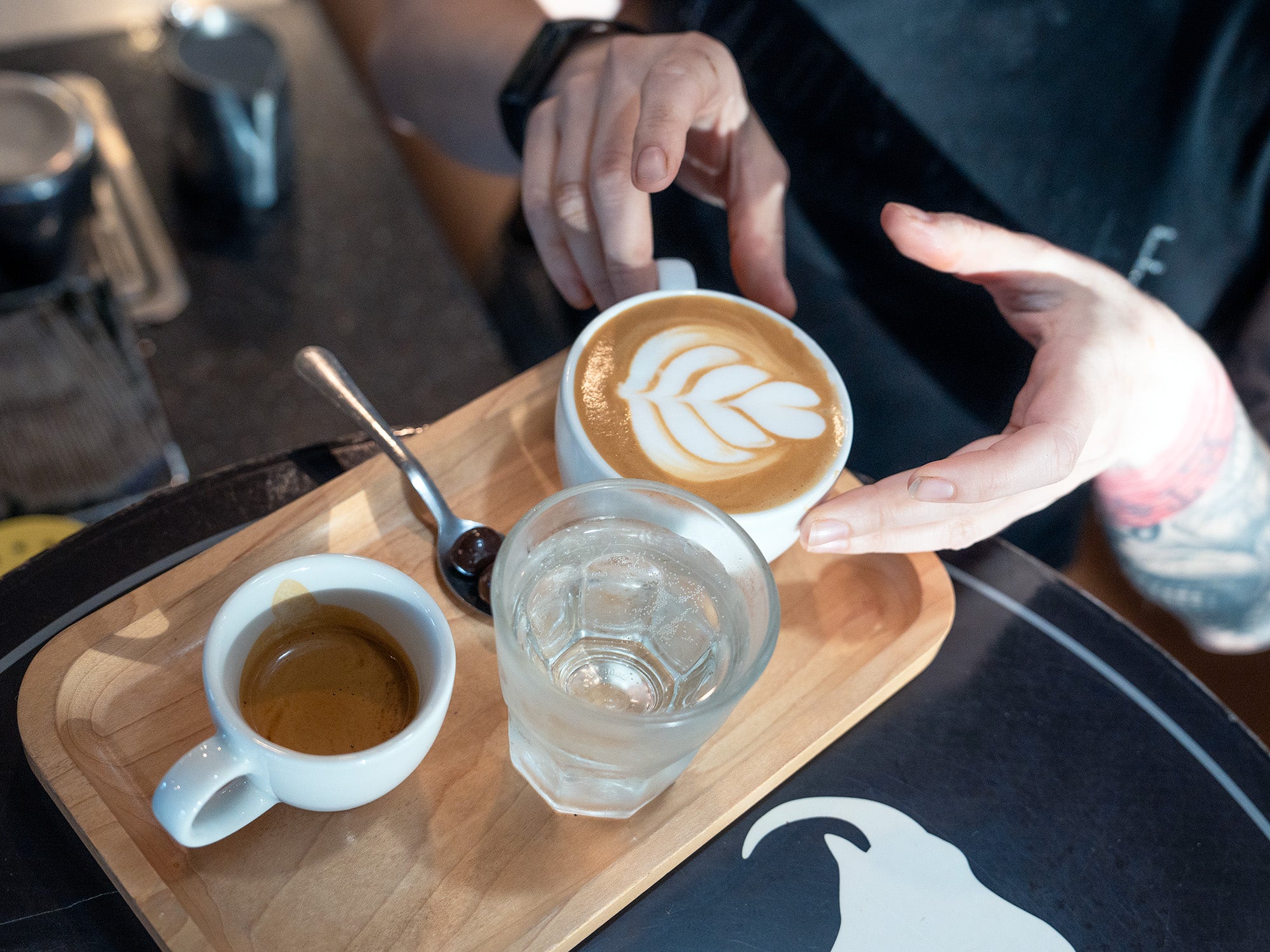In this detailed image, we see a close-up of a person with tattooed forearms reaching for a meticulously crafted latte. The caramel-colored coffee boasts an intricate floral latte art pattern with four swoops of white foam on its light brown surface. The latte sits on a small wooden tray located on a stylish black and white countertop. Accompanying the latte, to its left, is a glass of water containing a stirring spoon, and next to the glass is a small shot cup of espresso. The background is blurred, indicating the setting as a cozy cafe interior. This scene, rich in coffee culture elements, beautifully captures the moment of anticipation before savoring a perfect cup of coffee.